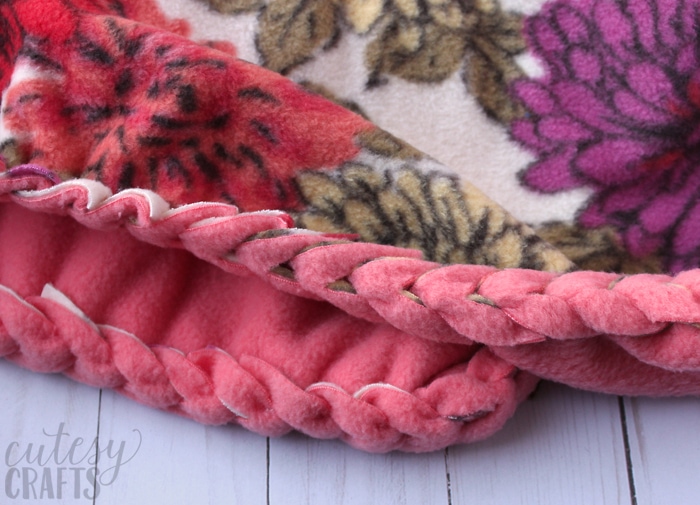The image showcases a detailed quilt sitting atop a slightly blue wooden table with visible gaps between its planks. The quilt, adorned with a thick braided border, features a predominantly pink hue interspersed with intricate red floral and purple leafy patterns. Additionally, it includes goldish-brown leaves set against a white background. The quilt conveys a sense of cozy craftsmanship, emphasized by its handmade, fleece-like texture and the whimsical, cartoonish design of the patterns. At the bottom left of the image, the text "Cutesy Crafts" is displayed, with "Cutesy" in cursive and "Crafts" in bold lettering, reinforcing the handmade and comforting aura of the quilt. The overall scene exudes a pastel, comfortable aesthetic, highlighted by the juxtaposition of the quilt's vibrant colors against the subtly purple-toned wooden table.